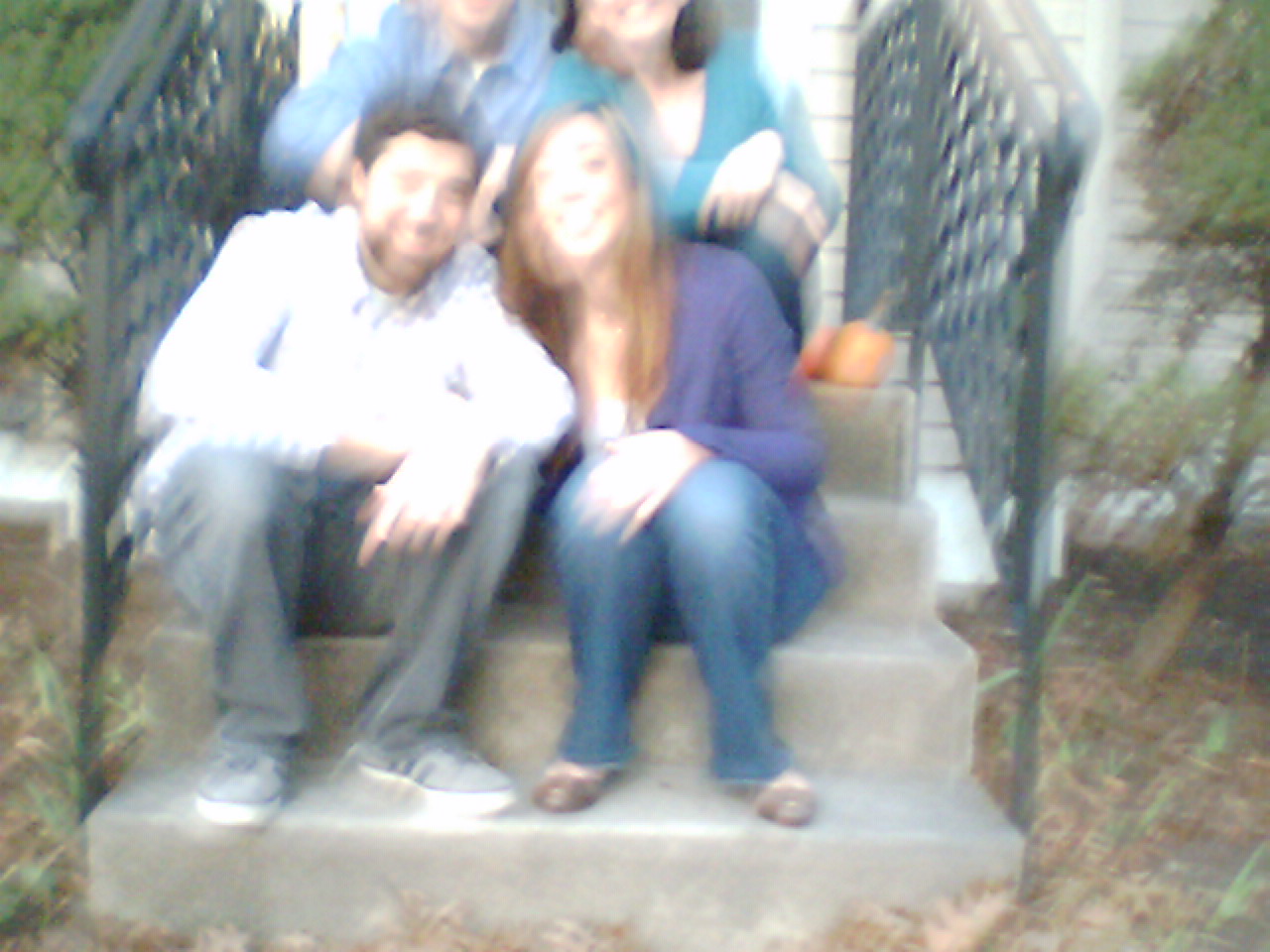A rectangular, slightly blurry photograph captures a moment of camaraderie among four individuals seated on a narrow set of light gray concrete stairs, consisting of four steps in total. The two people in the foreground are seated on the second step. On the left, a man is casually positioned with his elbows resting on his knees. He is dressed in gray pants, gray shoes with distinctive black stripes on the sides and white soles, and a long-sleeve button-up shirt. Next to him, on his right, sits a woman wearing a purple blouse layered over a white shirt, paired with blue denim jeans and brown pointed flat shoes.

In the background, on the fourth step, the two remaining individuals are partially cropped out of the frame, with only their torsos visible. The person on the left is clad in a blue button-up shirt, while the person on the right sports a blue v-neck style blouse. The photograph, although blurry, encapsulates a sense of casual relaxation among the group.